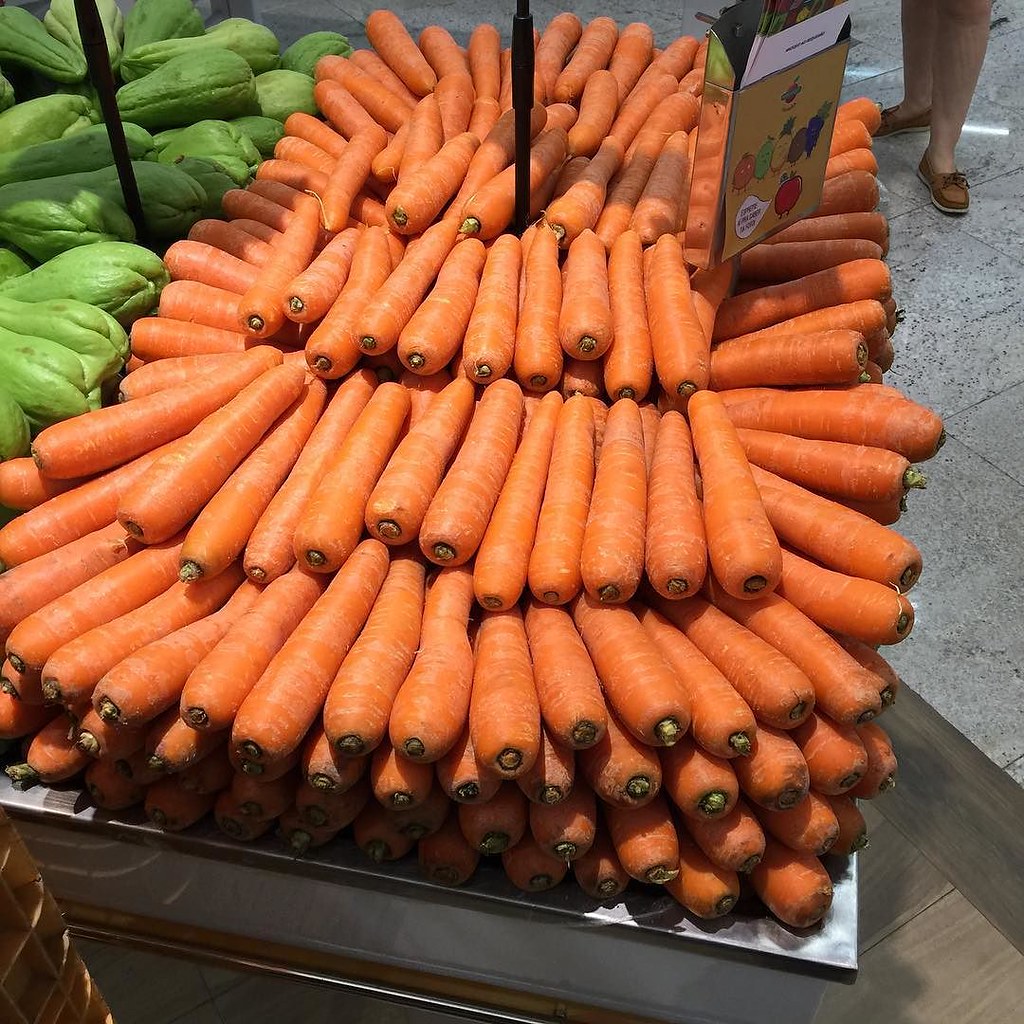This detailed image captures a vibrant scene likely set in an outdoor market, possibly an indoor Mercado. Central to the photograph is a meticulously organized display of large, unpeeled, and chunky carrots, predominantly stacked five layers high on a four-by-six-foot metal table. The carrots are arranged in a circular pattern with stems pointing outward and inward rows, creating an eye-catching centerpiece. To the left, a neighboring display of lime-green, possibly chayote vegetables, partly merges with the carrot arrangement.

The setting features a distinctive floor that transitions from gray tile with black details to vinyl wood, adding to the visual diversity of the scene. In the upper right corner stands a person, visible from the knees down, with light skin, wearing brown loafers or boat shoes without socks. A small, unreadable sign with animated vegetable cartoons and a yellow background is tucked among the carrots. Two black poles, potentially supporting overhead umbrellas, frame the display, enhancing the market ambiance. This lively snapshot provides a rich tableau of market life, brimming with fresh produce and subtle human presence.